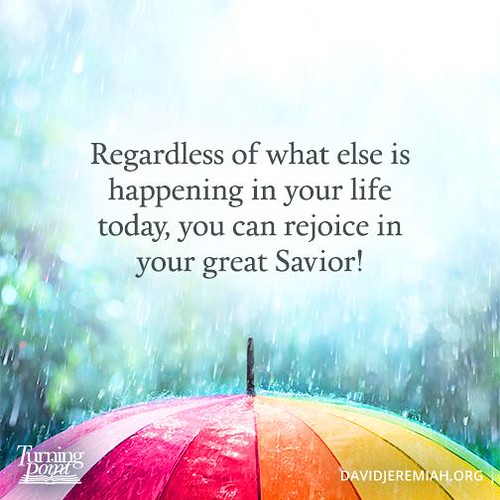This advertisement for the company "Turning Point" features a vibrant and eye-catching image of a multi-colored umbrella. The panels of the umbrella transition from pink, white, and purple on the left side to orange, yellow, and green on the right side, with a sharp white point extending from the top. Heavy rain is shown pouring down on the umbrella, creating splash effects that emphasize the downpour. The background is mostly blurred by a large white blur, but glimpses of raindrops and vegetation are visible behind it. Central to the poster, in bold black text, is an inspirational quote that reads, "Regardless of what else is happening in your life today, you can rejoice in your great Savior." At the bottom left corner of the image, "Turning Point" is written in white text, accompanied by a book emblem. The web address "davidjeremiah.org" is located in the bottom right corner, providing a clear call-to-action.